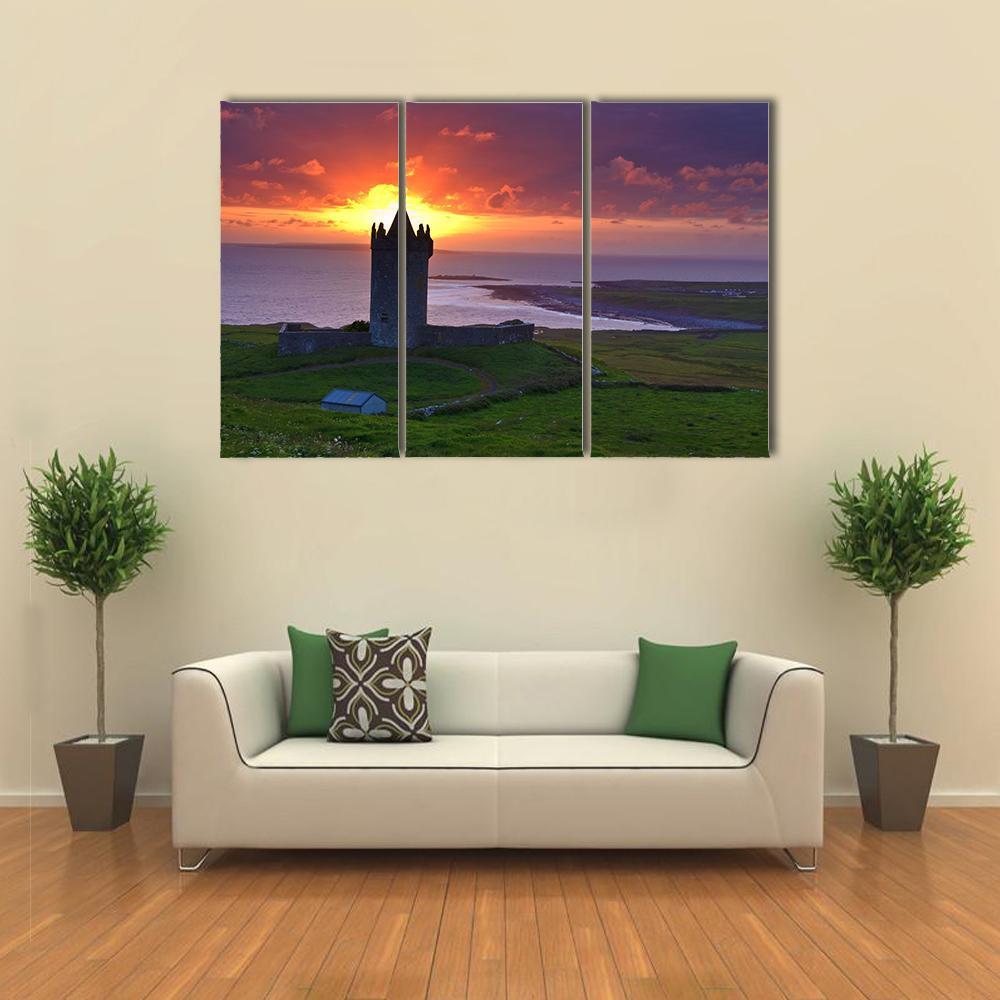This photograph captures a stylish living area featuring a beige wall and honey-brown hardwood flooring. Central to the space is a modern, cream-colored sofa outlined in black with short, silver hairpin legs. The sofa is accented by two solid green cushions in the corners, complemented by a brown and beige floral-patterned cushion placed in front of the left green cushion. Flanking the sofa are symmetrical small trees in square brown planters, adding a touch of greenery. Above the sofa, a striking triptych artwork commands attention, depicting a castle turret at sunset by a body of water. The vibrant scene features shades of purple, yellow, and gold in the sky, with lush green surroundings and a tranquil ocean or lake in the foreground.